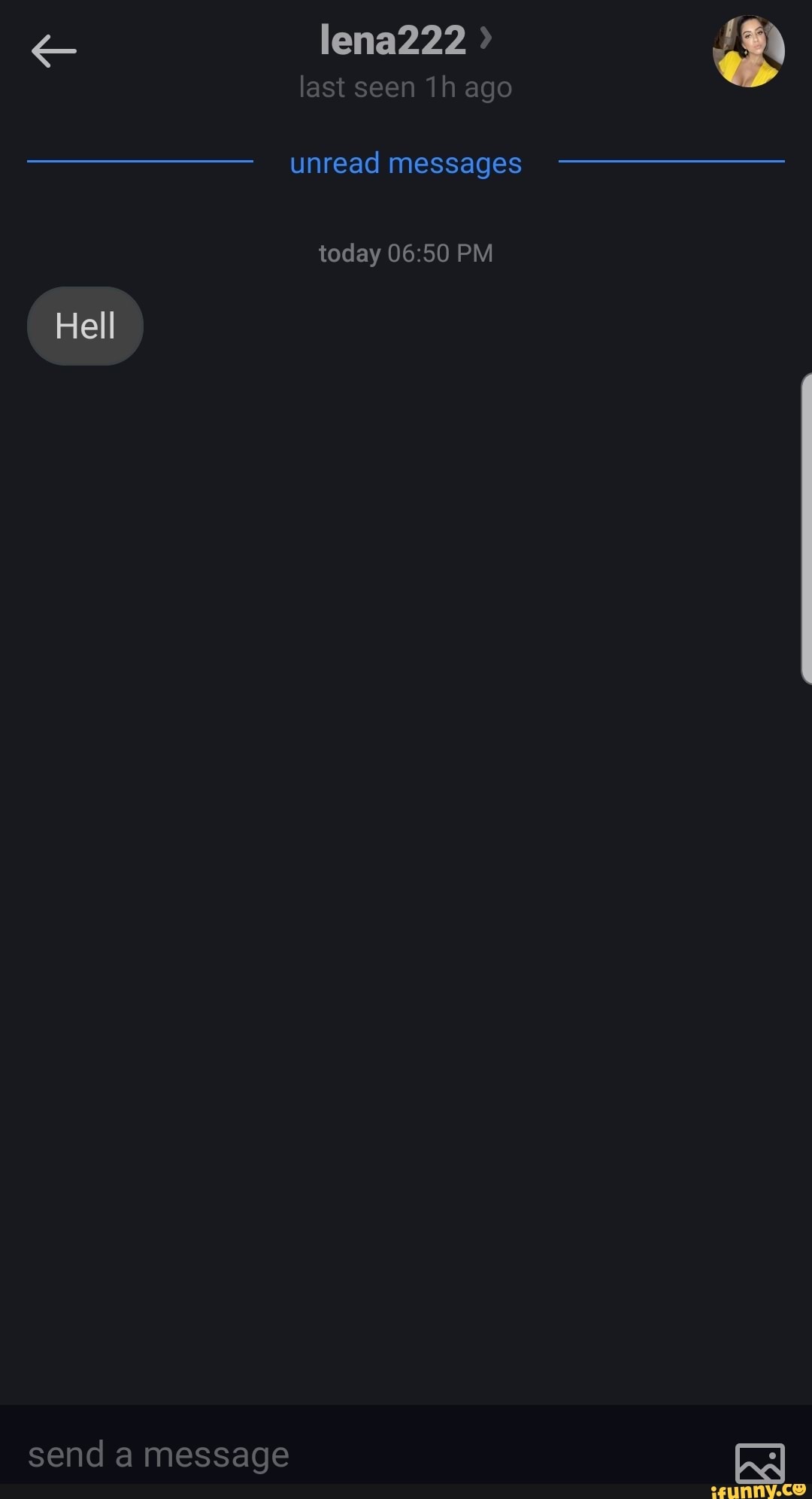The image appears to be a screenshot from a smartphone, depicting a messaging application's interface. The background is black. At the top of the screen, there is a light gray back arrow. Next to this, the name "Lina 222" is displayed in gray text, followed by a small right arrow icon in dark gray. Below this, also in dark gray text, is the status "Last seen one hour ago." On the right side of this header, there is a profile picture.

Below this header, a blue line divides the screen and includes the text "Unread messages" in the center. The timestamp "Today at 6:50 PM" appears in gray text beneath the blue line. Just below this, there is a gray message bubble containing the text "hell" written in white. 

A scroll bar on the right side indicates the screen is near the top of the conversation. At the bottom, a black section features the input field with gray text that says "Send a message," accompanied by a picture icon suggesting the option to share a photo.

There is a watermark at the bottom of the screen, partially cut off. It is in yellow and reads "iFunny.co," with the "o" resembling a happy face emoji.